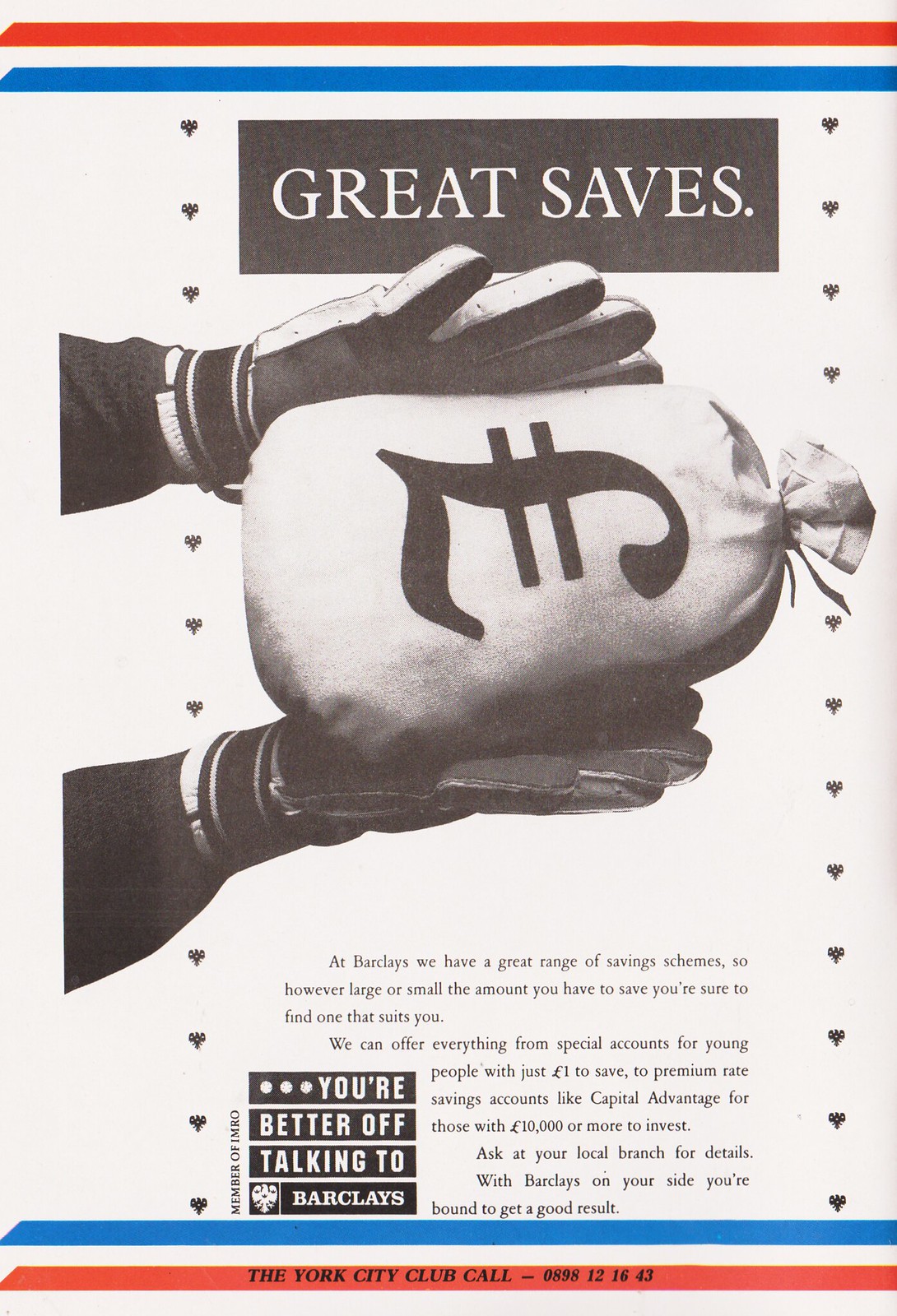The image is an advertisement on off-white paper, featuring a mix of black and white with a hint of red and blue accents. At the very top, a black box contains the phrase "Great Saves" in white font. Below this, there is a photograph in black and white of two hands wearing padded black and white gloves, holding a closed white bag marked with the pound (£) symbol. The hands seem to be demonstrating the idea of 'saving' money. Below the image, in small black font, the text reads: "At Barclays, we have a great range of saving schemes. So however large or small the amount you have to save, you're sure to find one that suits you. We can offer everything from special accounts for young people with just £1 to save to premium rate saving accounts with capital advantage for those worth £10,000 or more to invest. Ask at your local branch for details. With Barclays on your side, you're bound to get good results." The page also features horizontal lines in red and blue at the top and bottom. At the bottom, the text reads "The New York City Club" followed by a phone number, "Call 0898-121-643."